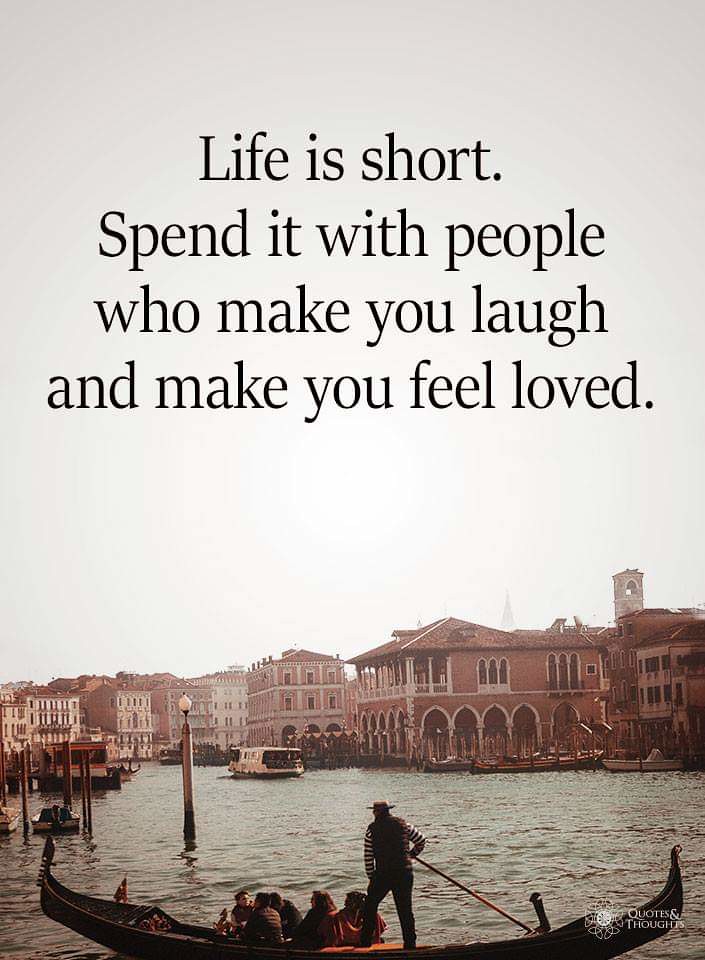The inspirational poster features a photograph likely taken in Venice, showcasing a serene canal scene. The image's upper half displays a clear, light gray sky, devoid of clouds. Prominently positioned across the sky is an inspirational quote in black text that reads: "Life is short, spend it with people who make you laugh and make you feel loved." Below, the canal is filled with several boats, with a focal point on a narrow gondola in the foreground. The gondola features multiple passengers and a standing gondolier, who is dressed in long black pants and a shirt with white and red striped sleeves. He is steering with a long wooden pole. The canal is lined with two-story buildings, enhancing the picturesque European ambiance. In the lower right corner of the image, there is a white text watermark that reads "quotes and thoughts."